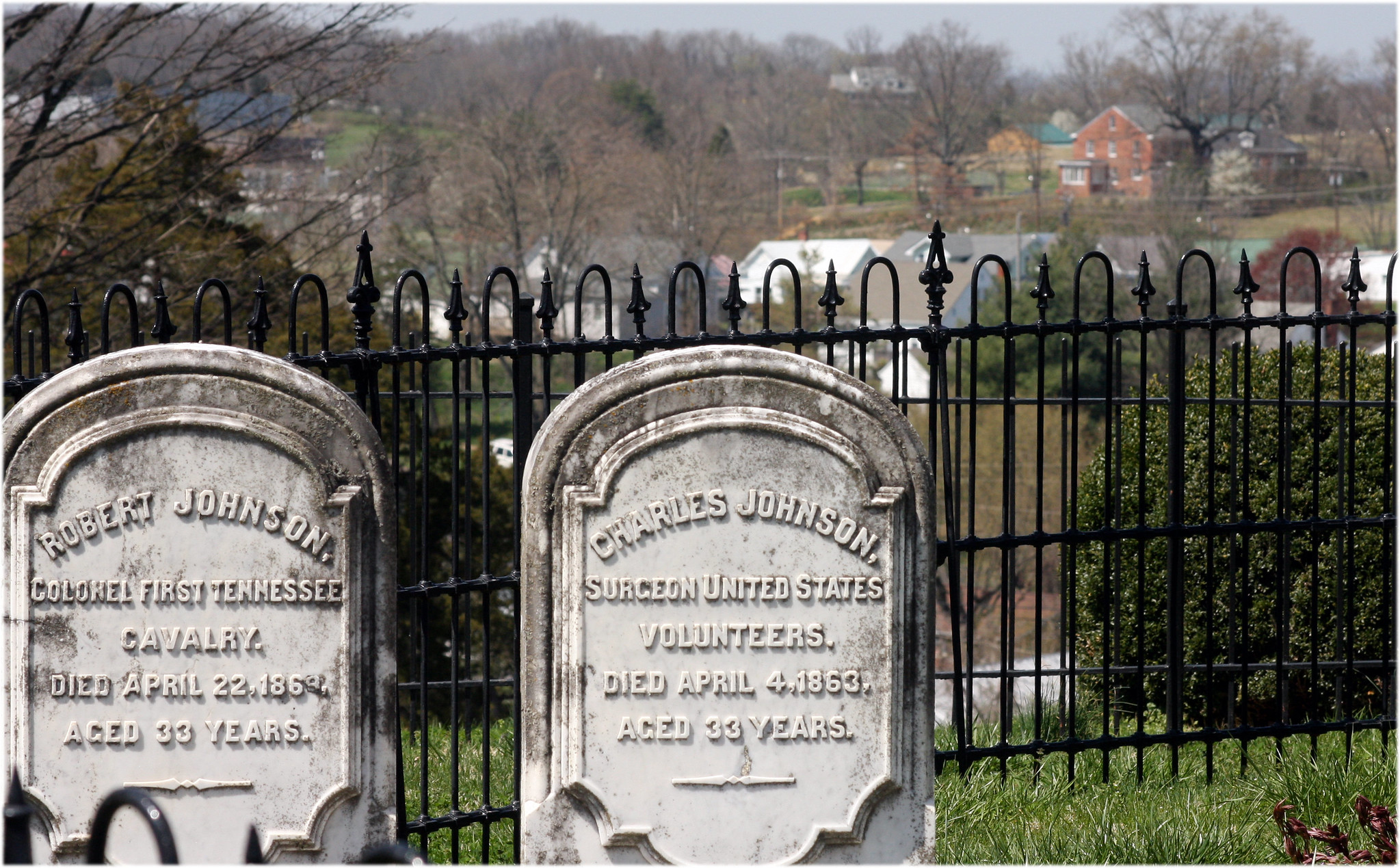The photograph captures a scene in an old cemetery, with two weathered, rounded-top gravestones made of stained concrete, prominently positioned in the lower section of the horizontal rectangular frame. The gravestones, adorned with decorative borders framing the engraved names and details, commemorate Charles Johnson, a surgeon who died on April 4th, 1860, at age 33, and Robert Johnson, a colonel in the First Tennessee Cavalry, who died on April 22nd, 1860, though the exact age is unclear. A black, decorative metal fence stands behind the gravestones, enclosing the space and marking a boundary.

The ground slopes gently downhill from the gravestones, leading into a grassy field interspersed with bushes and trees. The overall setting is an outdoor cemetery under a gray sky, hinting at a mid-day hour. Beyond the fence, a countryside landscape unfolds with a mix of buildings, including a farmhouse and other structures, some painted white with visible roofs. The horizon in the far background merges indistinctly, making it challenging to discern whether it is water or sky. The image is rich in color tones, featuring greens, browns, tans, oranges, yellows, grays, reds, and whites, all contributing to the serene yet somewhat somber atmosphere of the historic resting place.